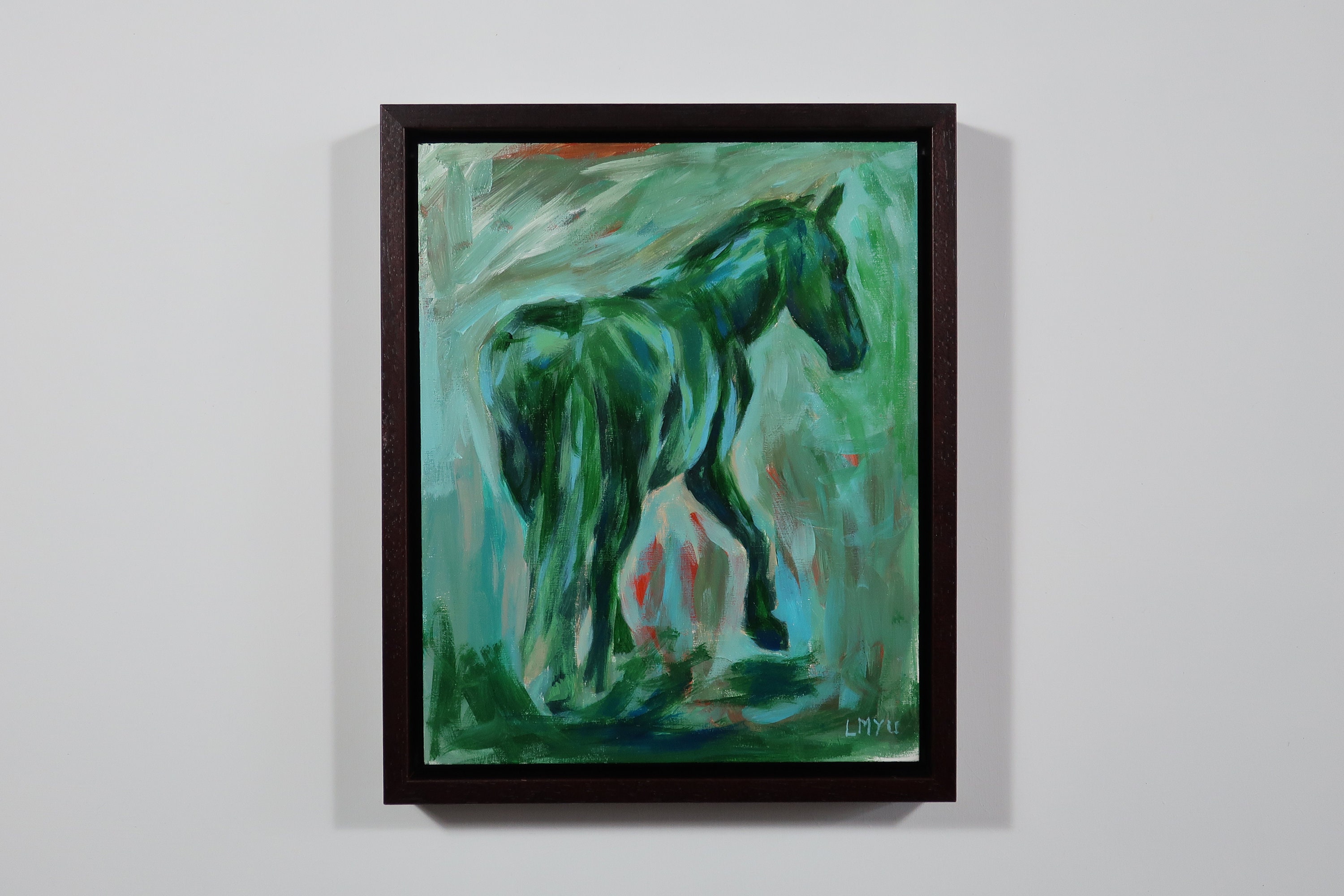This image depicts a framed, abstract oil painting of a horse positioned in the center of the canvas. The horse is facing away from the viewer with its tail and behind prominently visible, while its head is turned slightly to the right, giving the impression that it's actively walking. The frame is dark, possibly walnut wooden with a black border just inside it, and it encloses a smudgy composition of varying green and blue shades, including light green, dark green, turquoise, and light blue. Distinct red streaks and hints of black accentuate the abstract background, which suggests a grassy terrain with a sky containing light blue and dark gray tones. The artist's indistinct initials or name, "LMY" or "LMYU," are located in the bottom right, superimposed in a lighter blue color. The entire framed artwork is set against a dark gray background wall, providing a stark contrast that emphasizes the vibrant colors of the painting.